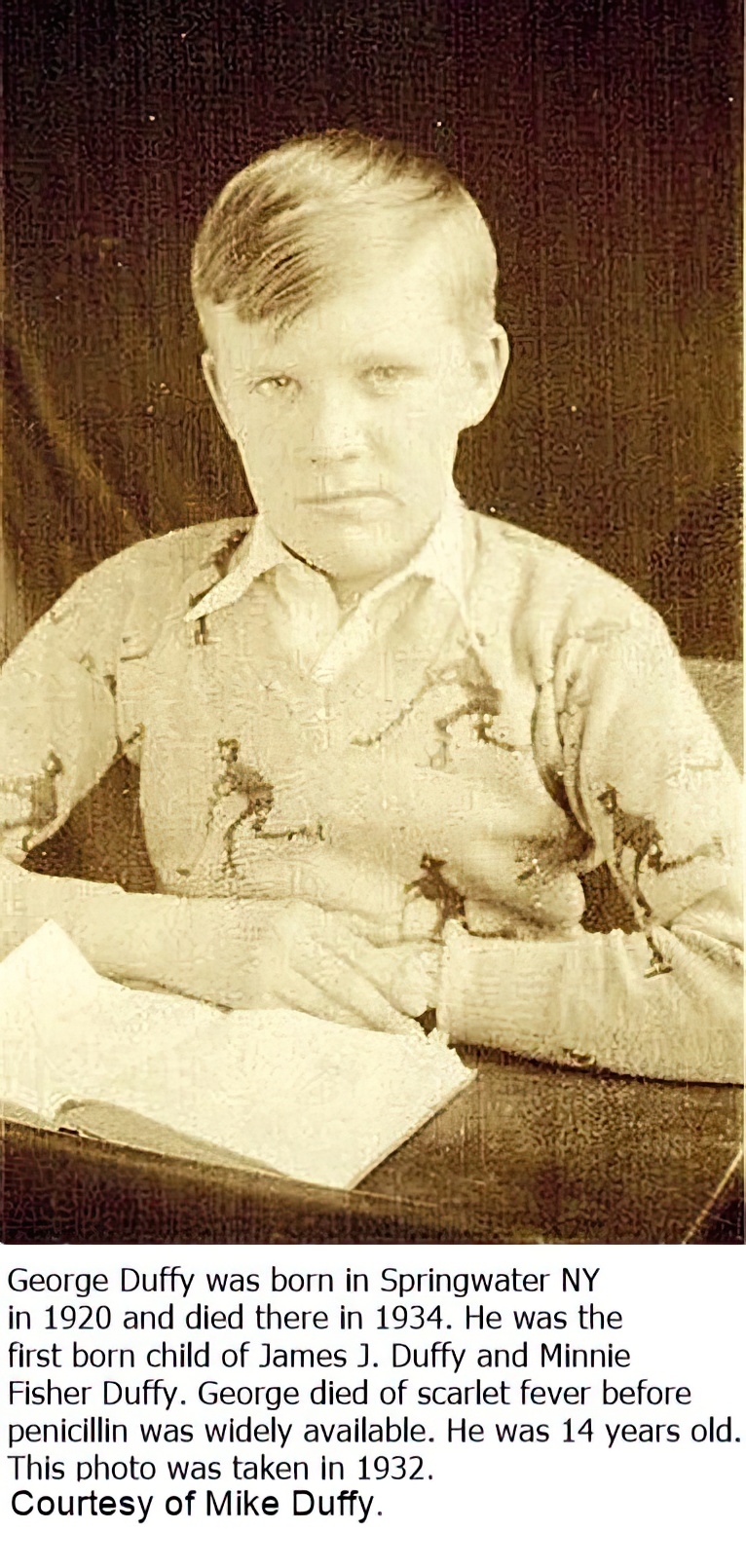This image is a faded, sepia-toned photograph of a young boy identified as George Duffy, who was born in Springwater, New York, in 1920 and passed away in 1934 at the age of 14 due to scarlet fever, before penicillin was widely available. The boy, with neatly combed hair, is seated at an empty wooden desk, arms crossed, looking towards the camera. He is dressed in a sweater adorned with images of hockey players, indicative of the style from the 1950s. An open book lies in front of him. The background is dark and appears to be cloth. The photograph is centered in the image with a black and white caption below it. The text reads: "George Duffy was born in Springwater, New York in 1920 and died there in 1934. He was the firstborn child of James J. Duffy and Minnie Fisher Duffy. George died of scarlet fever before penicillin was widely available. He was 14 years old. This photo was taken in 1932, courtesy of Mike Duffy."